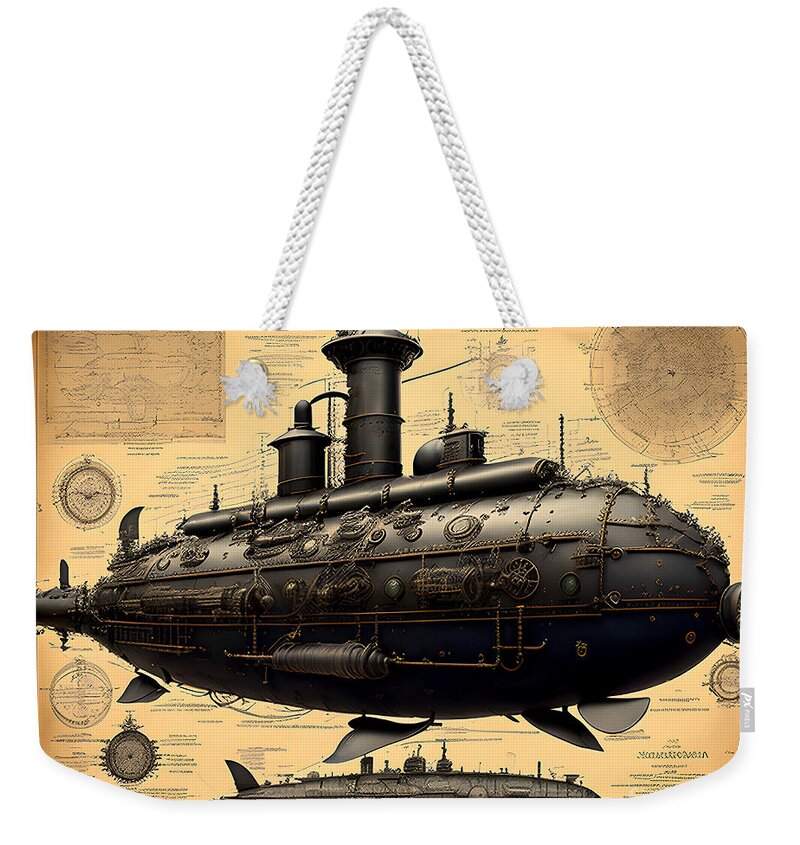This image depicts a detailed drawing of an early 1900s, rudimentary submarine. The artwork, with its old-fashioned aesthetic, showcases a dark gray, riveted steel submarine adorned with a multitude of mechanical elements such as gears, pipes, bolts, and small propellers. The submarine’s design is reminiscent of early steam engines, characterized by its robust and thick metallic structure. The background presents a cream-colored schematic chart filled with intricate diagrams and tiny, mostly illegible text in various fonts, adding to the technical and historical feel of the piece. The artwork is framed in an unconventional rectangular shape, with curved or trimmed edges on the bottom and sides, and is suspended by a knotted, braided rope affixed to the top, designed presumably to hang on a wall or display. The image appears on a handbag, against a bright yellow background, further accentuating the submarine and its detailed components.